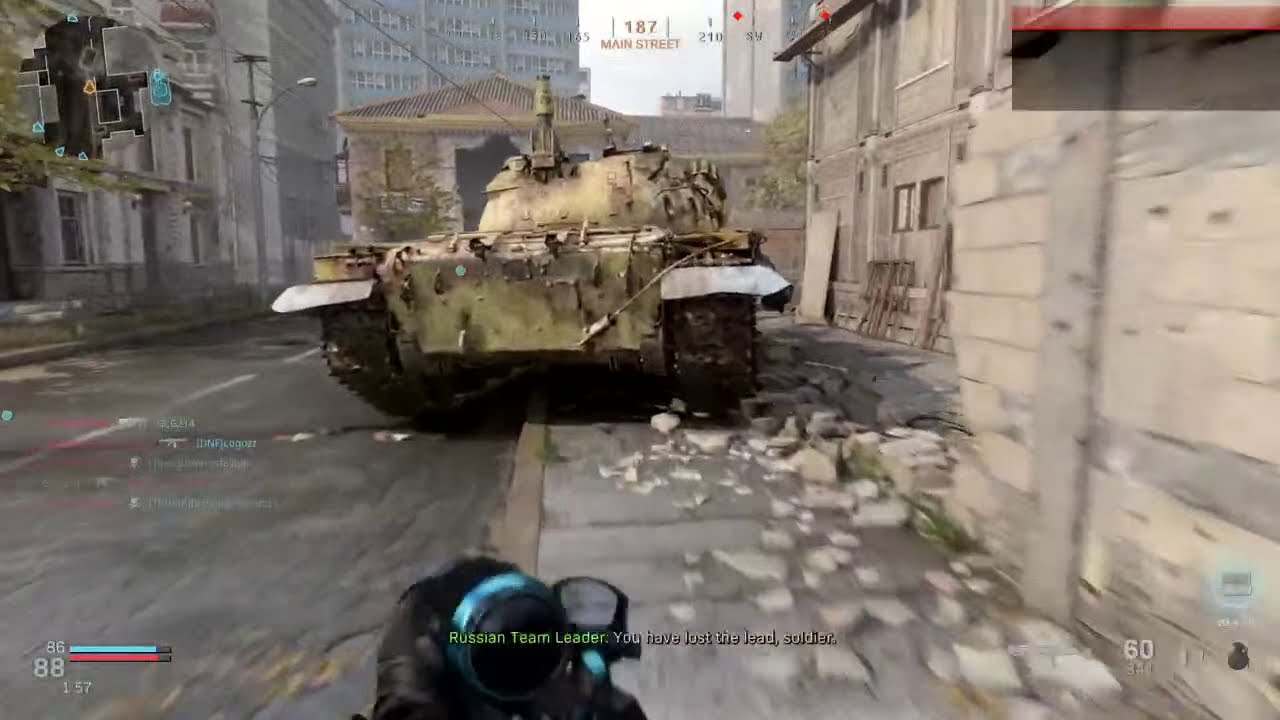The image is a detailed screenshot from a first-person shooter video game, depicting a war-torn urban setting. In the center, a large yellowish-brown tank is partially positioned on a street and partially on a concrete curb or sidewalk. Surrounding the tank are destroyed, burned-out buildings, resembling a devastated neighborhood, potentially in a European country. In the distance, a skyline of damaged buildings, including a skyscraper, can be seen.

The game’s Heads-Up Display (HUD) information is also visible. At the top, there's a compass rose indicating the player is facing 187 Main Street. In the upper left corner, a mini-map shows the player's position in orange and their teammates in blue. At the bottom center, text reads “Russian Team Leader. You have lost the lead, soldier,” indicating in-game communication. The bottom left displays the player’s health bar and stats, while the bottom right shows the ammo count and available lethals, like a grenade. The perspective includes the character's hand holding a gun, solidifying this as a first-person shooter game. The overall color palette includes various shades of gray, green, white, blue, red, black, and tan, enhancing the gritty and realistic war zone atmosphere of the game.